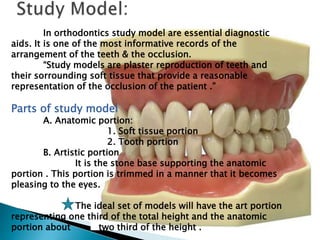The PowerPoint image showcases an essential educational tool in orthodontics, prominently titled "Study Model" at the top left. The text emphasizes the diagnostic importance of study models, describing them as plaster reproductions of teeth and their surrounding soft tissue. These models offer a comprehensive representation of a patient's occlusion, detailing the arrangement of the teeth. The background features a detailed model of human teeth, highlighting both the upper and lower portions, with pink soft tissue areas. The description further breaks down the study model into two main parts: the Anatomical Portion, which includes the soft tissue and tooth portions, and the Artistic Portion, represented by the stone base. This base is meticulously trimmed to be aesthetically pleasing, ideally with the artistic portion making up one-third of the total height and the anatomical portion two-thirds.